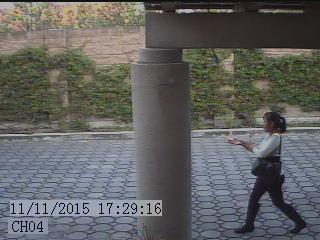The still frame, likely from a surveillance camera with the timestamp "11-11-2015 17:29:16" and labeled "CH-04," captures a scene where a woman is walking from right to left. She is dressed in a white long-sleeved shirt, black pants, and long black boots, with a black handbag slung over her left shoulder and her dark hair tied in a ponytail. She has her hands extended in front of her, as if carrying or rubbing something. The setting features a large gray cement pillar supporting a concrete roof at the center, and she walks on a gray cobblestone-like concrete pavement made of circular bricks. Behind her, a wall composed of brown stone with gray round pillars is partially obscured by green ivy vines. In the upper left corner of the image, some flowers are visible behind the wall.